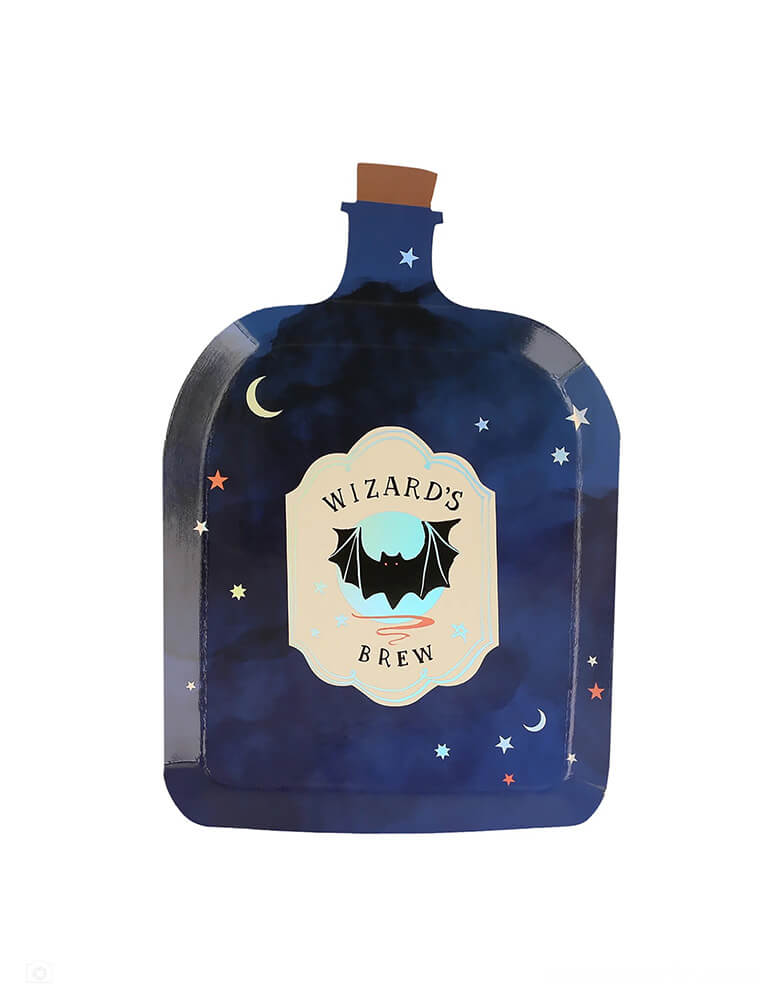The image is a detailed, colorful drawing or painting of a glass flask against a white background. The bottle is predominantly blue, with darker wispy cloud-like patterns on its surface, giving it a 3D appearance. Prominently displayed on the peach-colored label in all capital black letters is the text "Wizard's Brew." The center of the label features a cute, cartoonish black bat with orange eyes set against a blue circle. Scattered across the bottle are various star and moon designs, incorporating a soft blue and light beige color for the crescent moons, with some stars in red and white. Topping the bottle is a brown cork, completing the mystical and whimsical look of the "Wizard's Brew" flask.